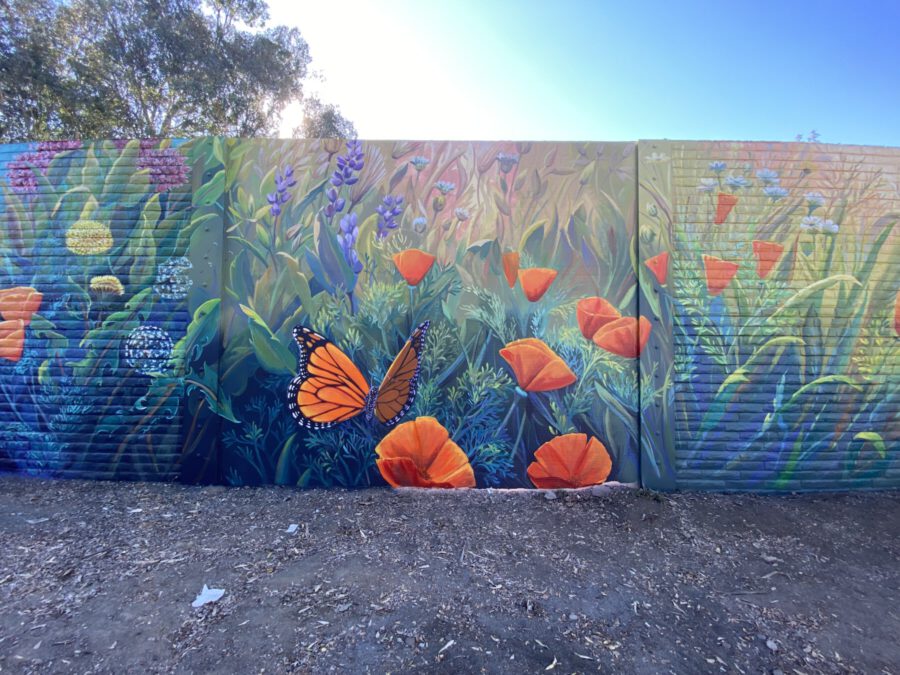This vibrant outdoor photograph, taken on a bright and sunny day under a blue sky, captures a colorful mural painted on a three-panel wall. The mural showcases an array of vividly depicted flowers and foliage, using a primary palette of orange, purple, and blue, with additional accents of yellow and green. The left panel features dandelions at various stages, with both blossoms and seed heads, set against a backdrop of purple and yellow flowers. The central panel highlights a striking monarch butterfly alighting on a red poppy, surrounded by green leaves and other purple and orange-hued flowers. The right panel continues the floral theme with more green foliage, small white flowers, and orange blossoms. Above the wall, the top of a tree is visible against the turquoise and blue sky. The mural is painted on what appears to be a mix of brick and smooth surfaces, possibly metal or wood, with the left and right panels showing a corrugated texture. In front of the wall is an area of dirt and dead leaves, which enhances the natural setting of this beautifully painted garden scene.